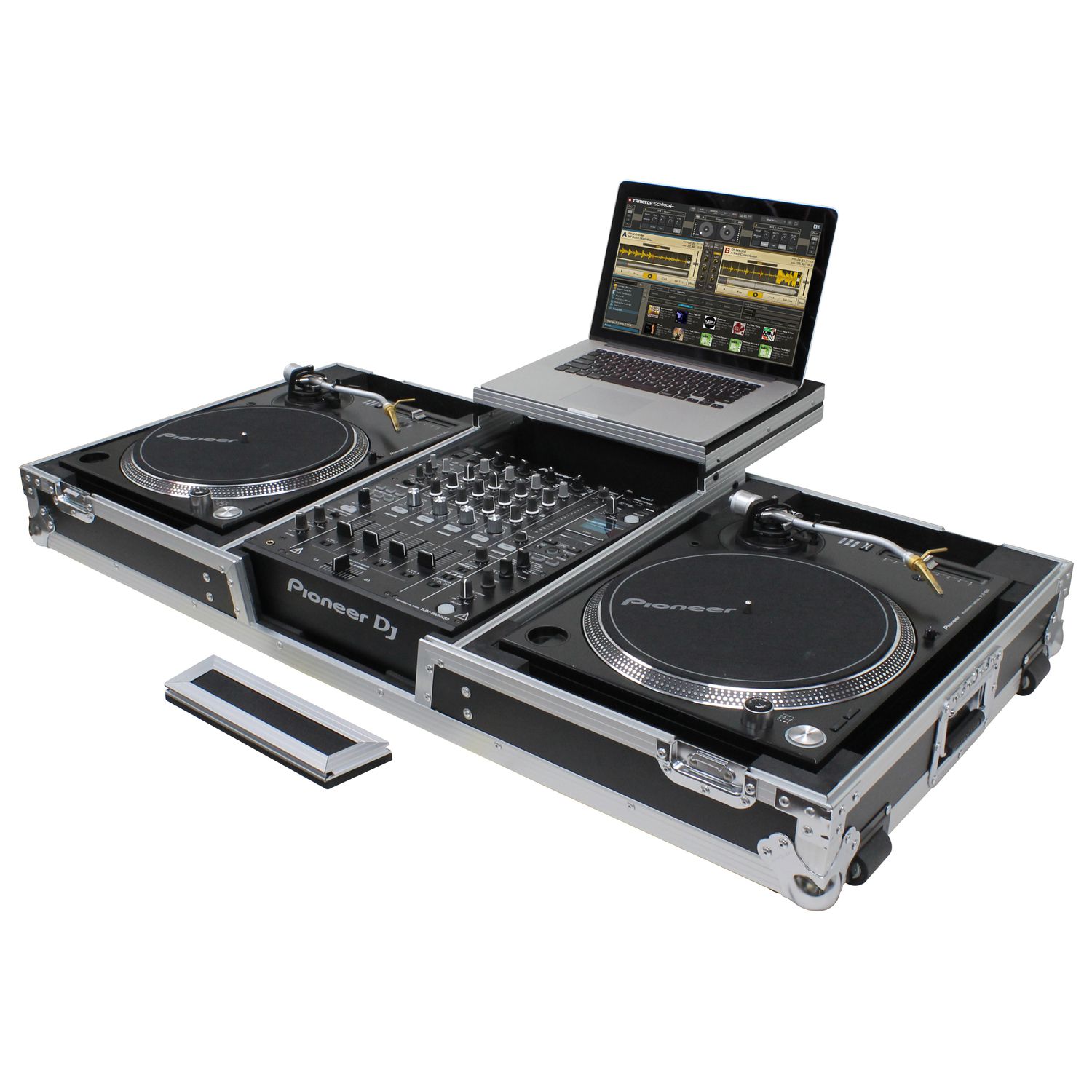This photograph captures a comprehensive DJ mixing system on a pristine white background. Dominating the setup are two turntables situated on the far left and right, perfectly designed for playing and scratching vinyl records. Centrally positioned between the turntables is an intricate control panel adorned with an array of knobs and dials for sound modulation and mixing. Prominently displayed on this control panel is the logo "Pioneer DJ" in gray against a black backdrop. Elevated behind this setup is a light gray laptop perched securely on a stand, its screen showcasing various music mixing programs and digital instrumentation, implying a direct connection to the DJ mixer. Additionally, in front of the mixing table but not attached to it, lies a small rectangular silver bar with a black center. This bar is possibly a stand or a resting aid for the DJ during mixing sessions.